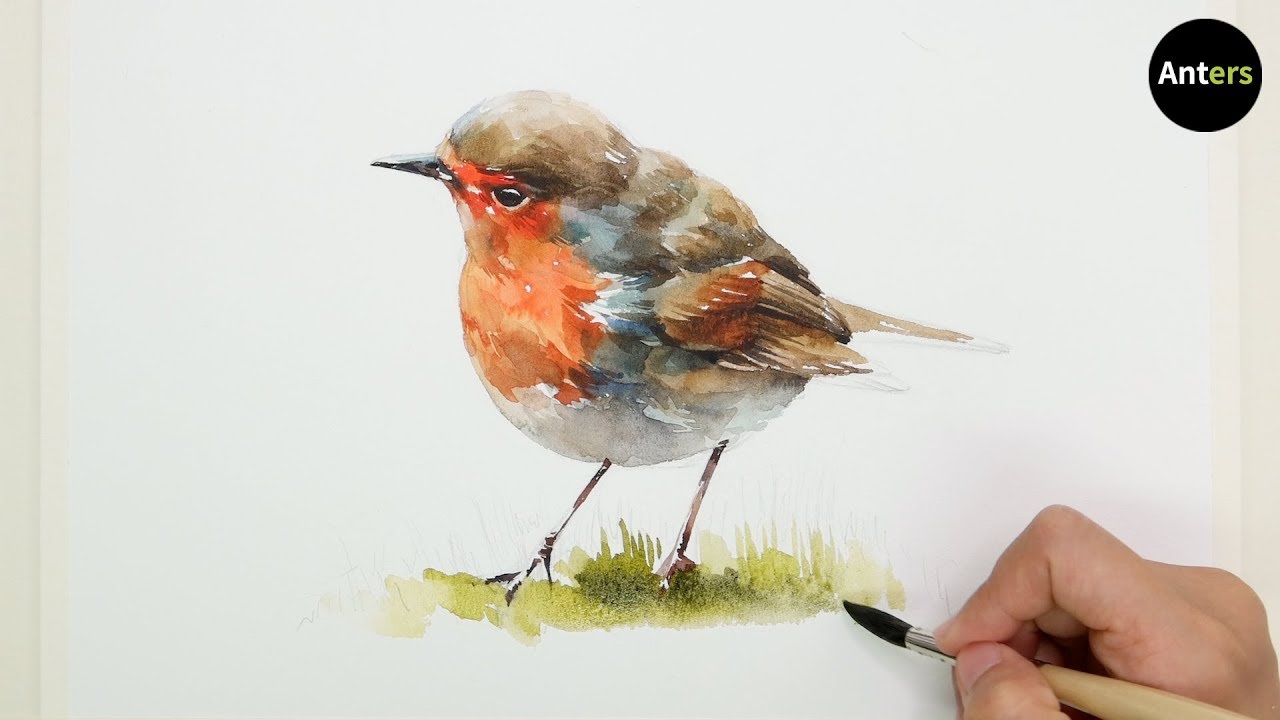The landscape-oriented photograph captures an artist's right hand in the bottom right-hand corner, holding a wooden paintbrush with a metal neck, actively painting a watercolor image of a robin bird. The partially visible hand touches up green grass beneath the bird's feet. The robin, facing left, features a dark brown back, a bright orange face and throat, with additional hints of orange on its wings. Its sturdy, yet small, body contrasts with its thin legs and delicate, short, pointy black beak. The bird's eyes are small, black, and beady, while its underbelly is white with patches of grayish and slightly dark blue feathers where the wings meet the body. A logo in the top right corner depicts a black circle with the word "Anters," where "A-N-T" is white and "E-R-S" is green.